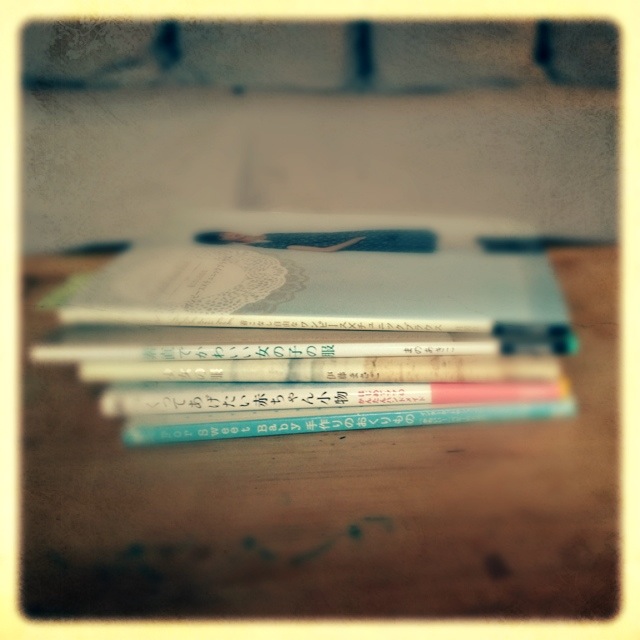The photograph is a slightly blurry color image capturing a stack of five thin books or magazines, all of which feature Chinese or Eastern lettering on their spines. The stack is centrally positioned on a brown wooden surface—possibly a table— with visible black marks in the foreground. The bottom left corner of the image is black, and the photograph overall has a yellow edge, giving it a Polaroid-like appearance. Behind the stack, there's a wooden wall with some visible bricks at the top. 

In the stack, the top book stands out with a pale blue cover featuring a large white circle containing illegible writing, and a photograph of a girl or woman with dark hair, dressed in a long blue dress and boots. The spines of the books are detailed: the first is yellow with a black line, the second is white with green letters and a black line, the third is yellow with gold letters, the fourth is white with black letters and a red bottom, and the fifth is light blue. Other notable colors on the spines include beige, dark pink, and sky blue. The overall dimension of the books suggests they are about the size of children’s reading books.